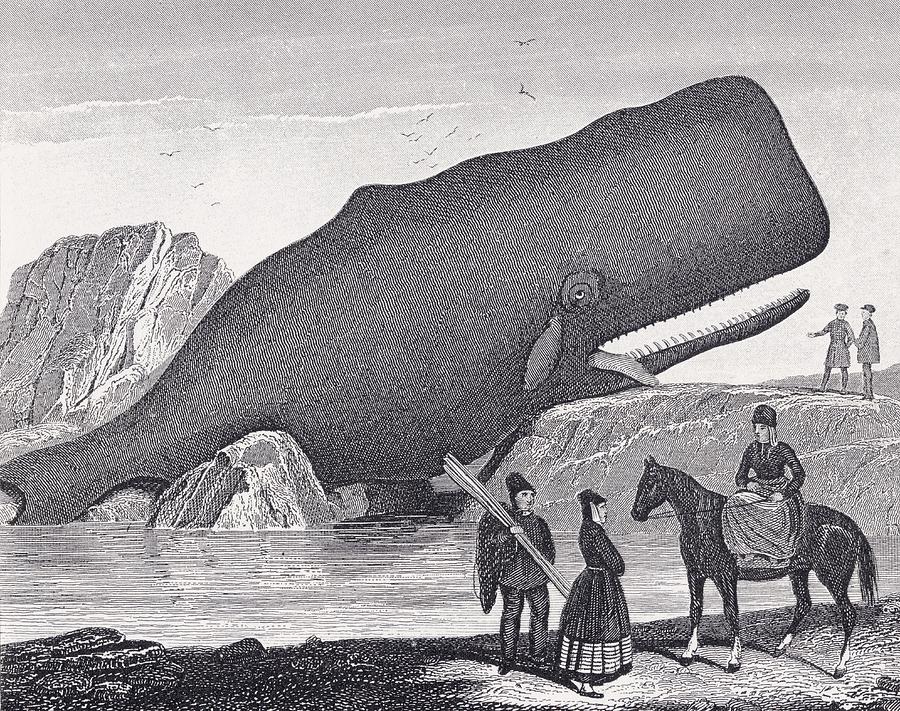The detailed illustration appears to be a pen and ink drawing, likely from the 1700s or 1800s. This black and white piece depicts a dramatic scene of a gigantic, deceased whale that has washed ashore onto a cold, rocky beach. The whale lies almost fully out of the water, positioned sideways with its mouth wide open, revealing numerous teeth and a protruding tongue, emphasizing its lifeless state. Beside the whale, on the rocky terrain, two men dressed in traditional Western attire are engaged in conversation, with one gesturing toward the enormous creature. 

In the foreground, a distinct group captures the viewer's attention: a man sitting side-saddle on a horse with four white socks, wearing what seems to be Asian dress, and two other individuals—one holding sticks and a woman in a dress—standing nearby, seemingly in discourse over the situation. Above, the sky is filled with seagulls flying around rock formations, casting a somber mood over the scene. The entire composition powerfully conveys a moment frozen in time, capturing both the tragic demise of the whale and the human reaction to this spectacular event.